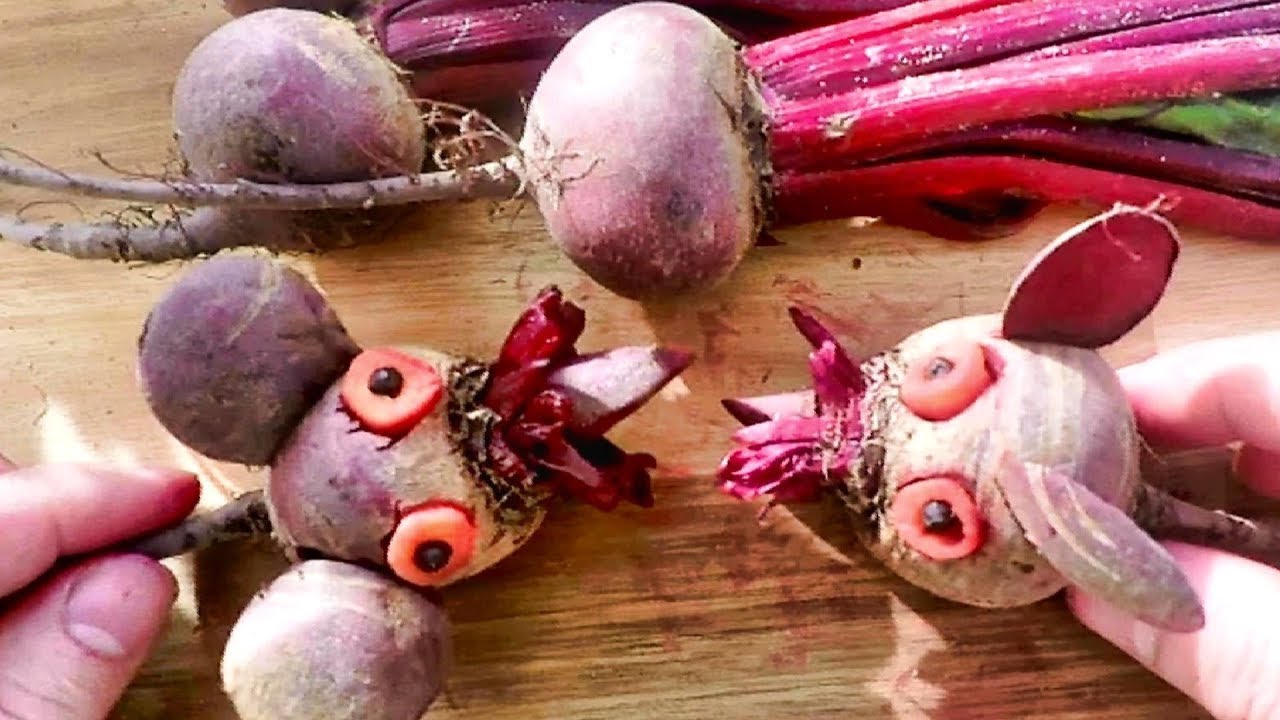In this image, a pair of white hands hold two intricately decorated beets on a light brown table, possibly in a home kitchen setting. The foreground beets have been transformed into whimsical characters, each featuring eyes crafted from carrot slices and ears made from beet slices. These creations face each other with charming expressions. Their hues range from a dark, toned-down maroon to a purplish-red. Some retain their roots, adding to their rustic appearance. The beets look slightly dirty, suggesting they were freshly picked. In the background, two additional unadorned beets, with attached roots and stalks that transition from dark purple to bright red and magenta, can be seen lying on the table.